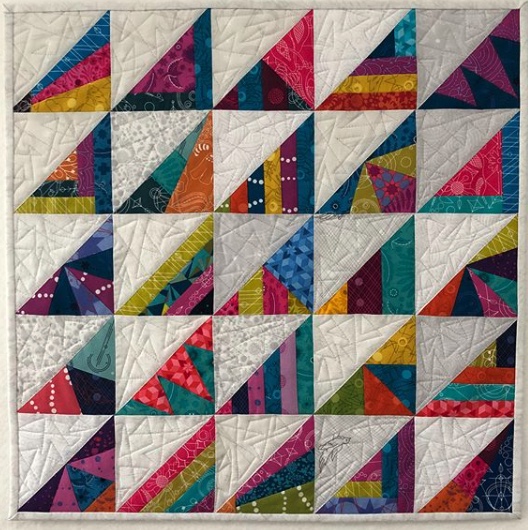This is an intricately designed quilt arranged in a square format with a five-by-five grid of patches. Each patch is divided diagonally from the bottom left-hand corner to the top right-hand corner. The upper left triangle of each patch features a uniform white fabric with subtle abstract stitching patterns. In contrast, the bottom right triangle of each patch is vibrant and varied, showcasing an array of colors and designs including blues, oranges, purples, yellows, and greens. Some patches have stripes, others have geometric shapes like squares and triangles, and a few feature tiny patterns of dots or abstract shapes. The quilt is bordered by the same white material found in the upper left triangles, adding a cohesive frame to the colorful and dynamic center design.